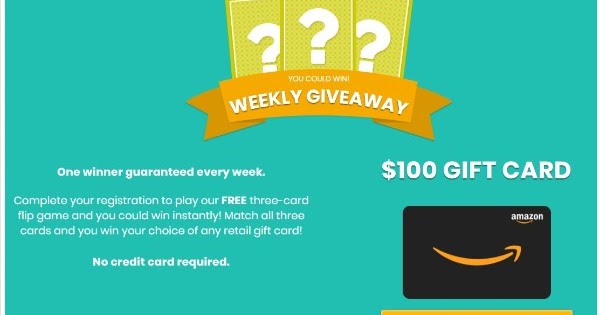**Caption:**

In the screenshot, we see a visually engaging game promotion set against a greenish-blue-teal background. At the top center, three green cards are displayed, each marked with a white question mark. The cards overlap slightly, with the central card overlaying the ones to the left and right. Below the cards, a goldish-orange banner features bold white text that announces, "You could win a weekly giveaway!"

On the bottom left-hand corner, white text explains the game: "One winner guaranteed every week. Complete your registration to play our free three-card flip game and you could instantly win. Match all three cards and you win a choice of any retail gift card. No credit card required."

To the right, the text "$100 gift card" appears prominently next to an image of a black Amazon gift card. The card features the iconic white Amazon logo in the upper right, accompanied by the distinctive smiley-face arrow stretching from the 'A' to the 'Z'.

Just below the Amazon card, a hint of an orange box is visible, though the contents are obscured and unreadable. The promotional image effectively entices viewers with its vibrant colors, clear instructions, and the promise of a valuable prize.